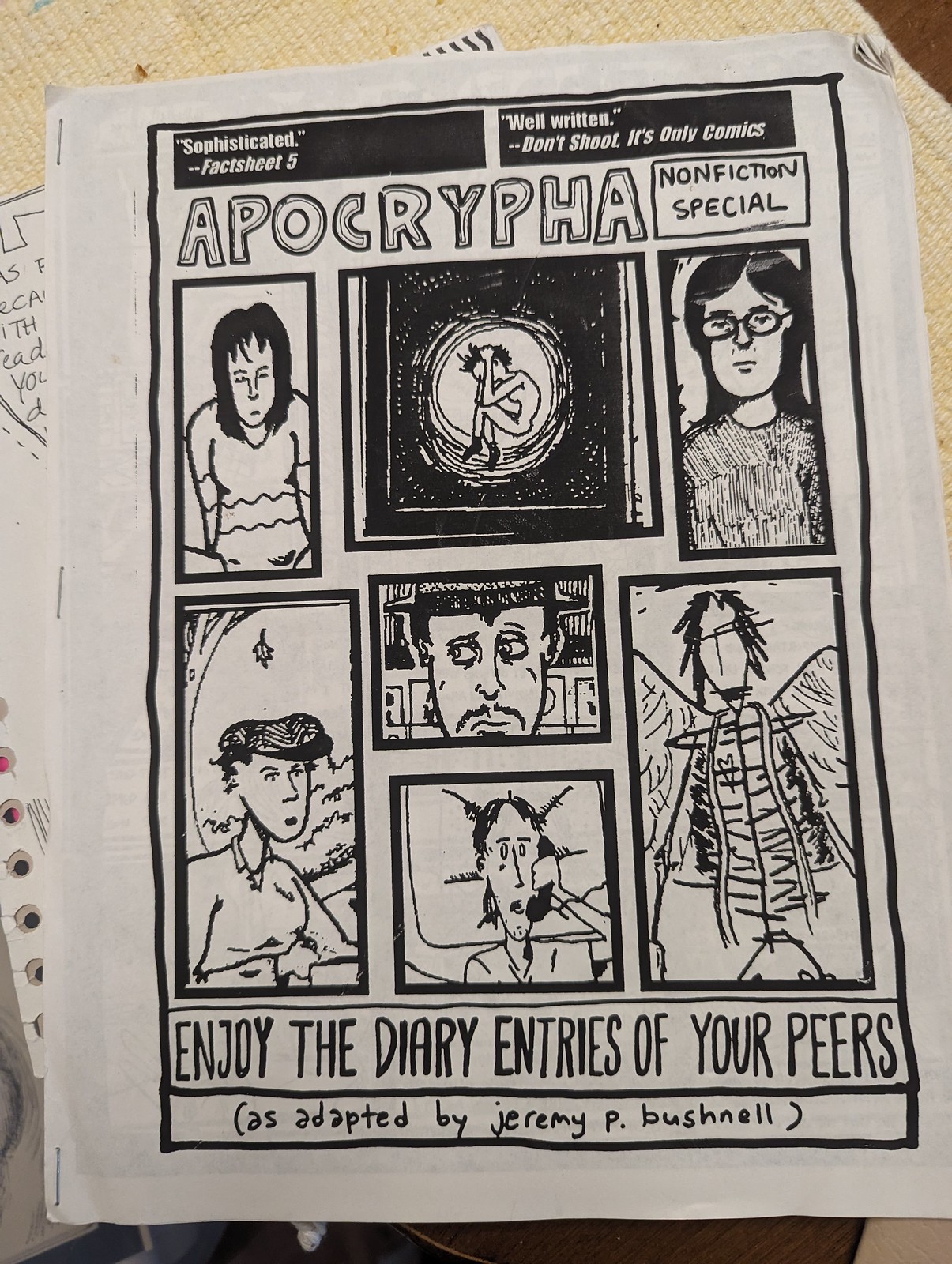The cover of the magazine or comic booklet, resting on a fabric surface, features a white sheet of paper bound together with three unevenly placed staples on the left side. The top of the cover flaunts a black rectangle with white text that reads "Sophisticated, Fact Sheet 5," and a white rectangle to the right with the words "Well Written, Don't Shoot, It's Only Comics." The prominent title, "Apocrypha," is displayed in white font with a black border. The cover is a mix of text and hand-drawn images, suggesting a handmade quality. There are seven different drawings, including a person with hunched shoulders in the top left, another person curled up in a ball in the middle top section, and an individual wearing glasses on the right. The booklet also mentions "Nonfiction Special," adding to its eclectic and detailed appearance.